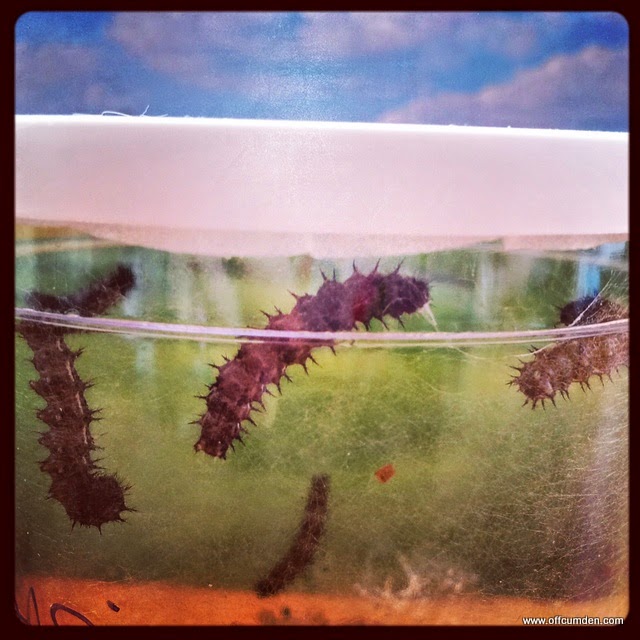The image showcases a close-up view of a transparent plastic container with a white lid and an orange bottom. Inside the container are four spiky, red-purple larvae or caterpillars, entangled in a web of white fibers. The background inside the container appears green, which, coupled with the larvae and web, gives an impression of greenish liquid that might actually be an optical illusion. The container is framed by a light blue sky with clouds at the top of the picture. The entire image is enclosed in a black frame, and in the lower right corner, the website "www.afkandom.com" is prominently displayed.